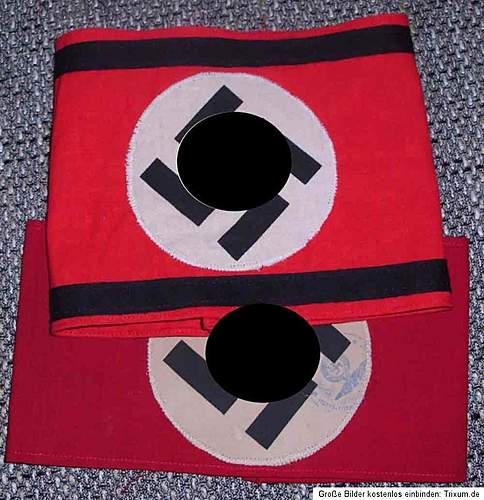This is a staged, full-color close-up photograph taken indoors, possibly on a mat or tablecloth with a black and white repeated pattern. The image centers on two old Nazi armbands. Each armband is red with a white circle in the middle, containing a black swastika, which has been censored with a black dot. The smaller armband, with lighter red and black bars on the top and bottom, contrasts with the larger, darker red armband that lacks these additional black bars. At the bottom of the image, text reads, “Grobe, Builder, Kostenlos, Einbinden, Trixum.de.” The overall image evokes a disturbing view of this Nazi memorabilia.